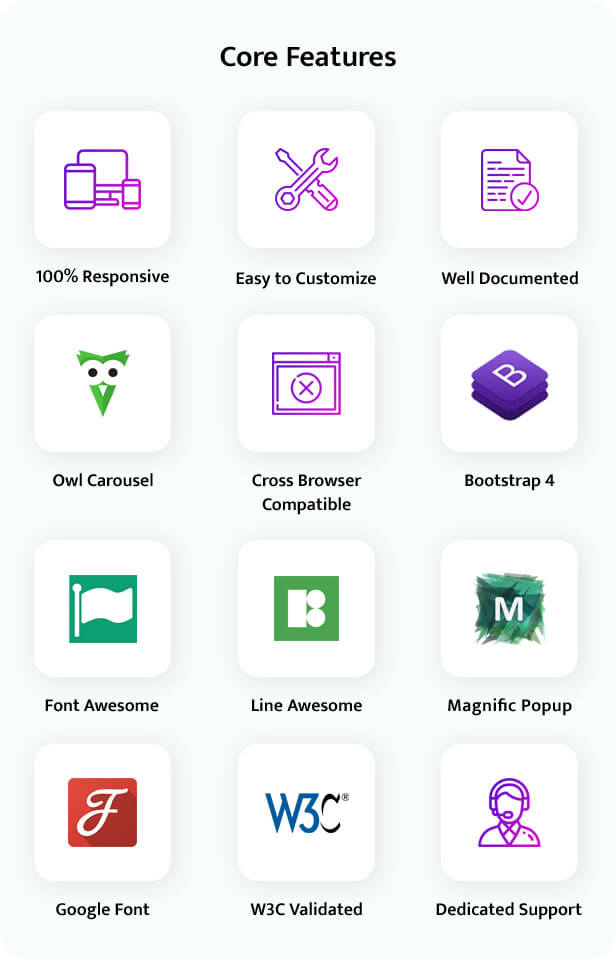This image showcases the core features of a product, possibly a mobile application or a website, clearly organized in a layout that resembles the dimensions of a phone screen. The central part of the image prominently highlights these core features. Each feature is depicted with icons encased in selection boxes.

Starting from the top left, the first icon is that of a computer, and below it, the text reads "100% Responsive," indicating the product's compatibility across various devices. Adjacent to this is an icon of a wrench, symbolizing "Easy to Customize," which suggests user-friendly customization options.

To the right is an icon of a document with a checkmark, labeled "Well Documented," hinting at comprehensive and accessible documentation. Below this first row is a second row of icons, starting with a carousel indicating the product is "Cross Browser Compatible," ensuring functionality across different web browsers. Next to it is the logo for "Bootstrap 4," signifying the use of this popular front-end framework.

The following line starts with an icon indicating "Font Awesome," a library for scalable vector icons, followed by another icon representing "Line Awesome," a similar icon toolkit. The next icons represent "Magnific Popup," a lightbox plugin, "Google Fonts" for typography options, "W3C Validated," indicating standards compliance, and "Dedicated Support," which promises user support services.

While some icons are just outlined in purple, giving them a minimalistic look, others are more colorful, likely signifying their more significant impact or association with respective companies. The combination of outlined and colored icons provides a visually appealing contrast while effectively communicating the product’s features.